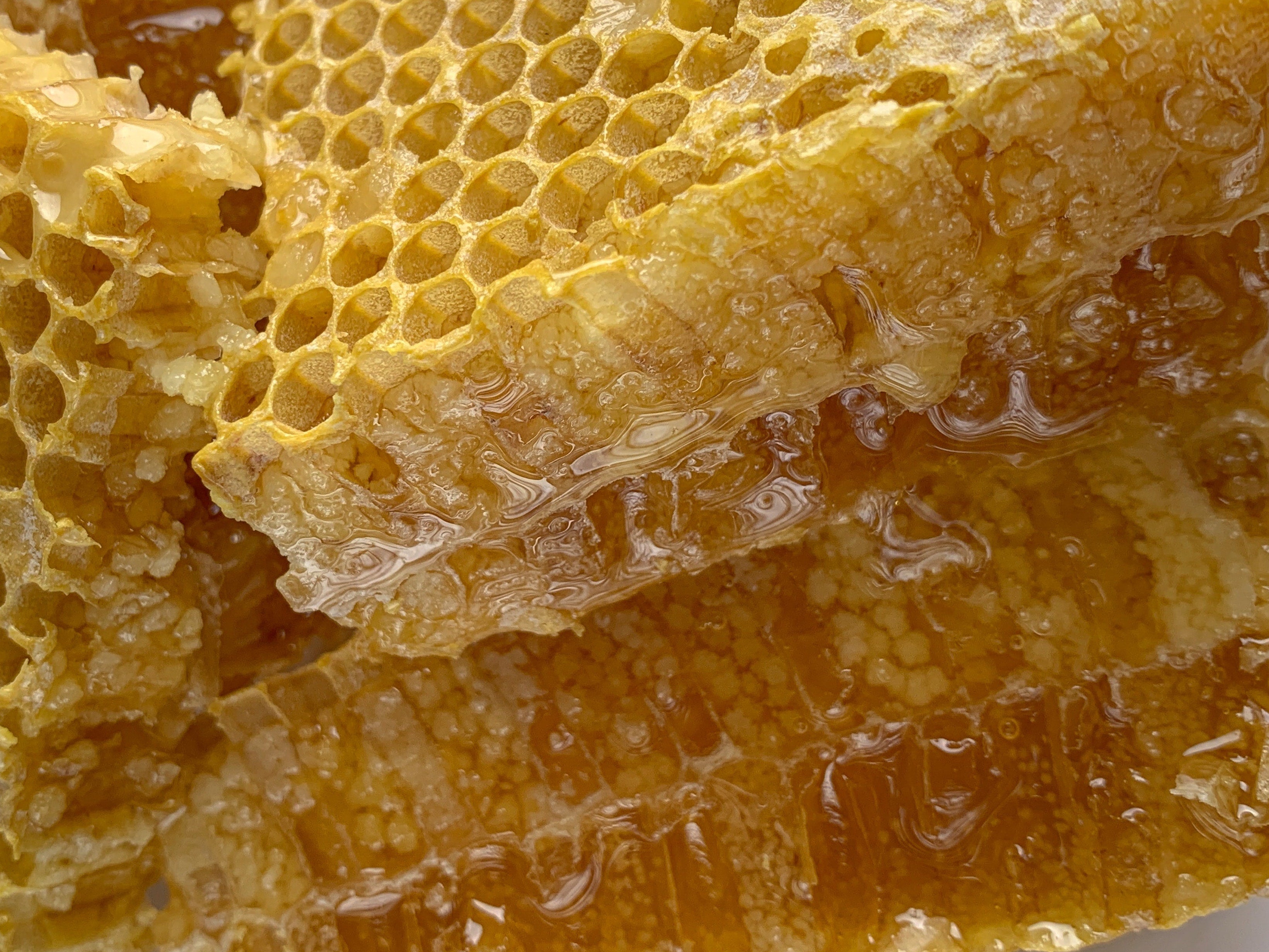This highly detailed and zoomed-in photo captures multiple pieces of honeycomb, intricately showcasing their texture and vibrant hues. The honeycomb, appearing waffle-like with its uniform holes, is predominantly a golden yellow, while the honey itself takes on a darker yellowish-orange tint in some parts. The combs are arranged in what appears to be stacked, square-ish shapes, and one piece on the left is broken open, revealing the inner texture. The topmost comb is laid flat, allowing a view into the sides of its holes, though the depth of the holes is not visible from this angle. Honey is both crystallized and liquid, shimmering under the light, and visibly dripping off the lower sections, giving the image an overall wet and sticky appearance. The white palette in the background is barely visible at the bottom right corner, emphasizing the honeycomb's rich colors and textures. The photograph's exceptional detail, aided by high-quality lighting and lens, captures the honey's fluidity and the comb's structural intricacies perfectly.